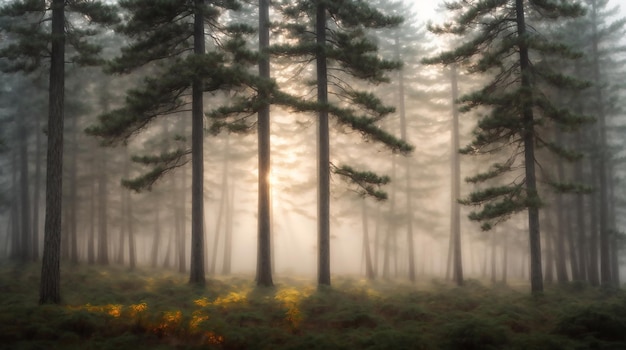The image, taken outdoors in daylight, depicts a serene forest scene that almost resembles a painting. Tall, mature pine trees, reminiscent of Christmas trees or lodgepoles, dominate the landscape, flanking both sides and culminating in a trio of prominent trees standing side by side in the middle. The forest floor is covered in overgrown grass, dotted with different plants and flowers, including some with yellow petals and hints of orange in the bottom left corner. The misty, almost foggy atmosphere softens the background trees, creating a sense of depth and tranquility. Sunlight pierces through the trees, casting dappled light on the foliage below and revealing a faint glimpse of the white sky above. The interplay of light and shadows, combined with the subtle morning mist, lends the forest a magical, ethereal quality.